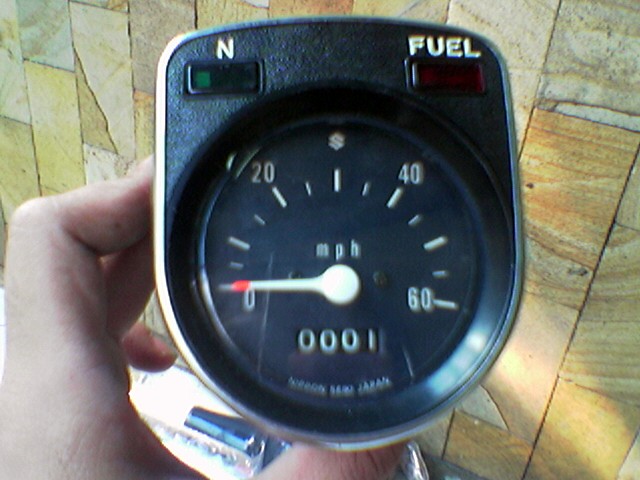In this slightly blurry image, a man is seen holding a distinctive speedometer-like instrument in his left hand. His thumb is positioned underneath the device, centered at the bottom, while his fingers grip the side securely. The instrument itself has a unique design, being square at the top and round at the bottom. It is predominantly black but features a silver outline that encompasses both the top and the entirety of the device.

In the top-left corner of the instrument, there’s a small rectangular green indicator light. Adjacent to this, on the right side, a capital 'N' is prominently displayed in white. Below this, another small rectangular indicator in red is clearly labeled 'fuel.' Dominating the center of the device is a circular speedometer face. The top of the speedometer is adorned with the Suzuki logo, represented by a simple 'S.'

The speedometer scale ranges from 0 to 60 in a semicircular layout, with a white dial to indicate speed. Just above the dial, 'MPH' is inscribed in small letters. Within the circular display, there’s a rectangular panel that shows the number '001.' At the very bottom of the circular face, small curved white text adds a final touch of detail.

The background features a child-height stone wall, providing a contrasting backdrop to the held instrument. This combination of elements ensures the viewer's focus remains on the intricate details of the speedometer device the man is presenting.